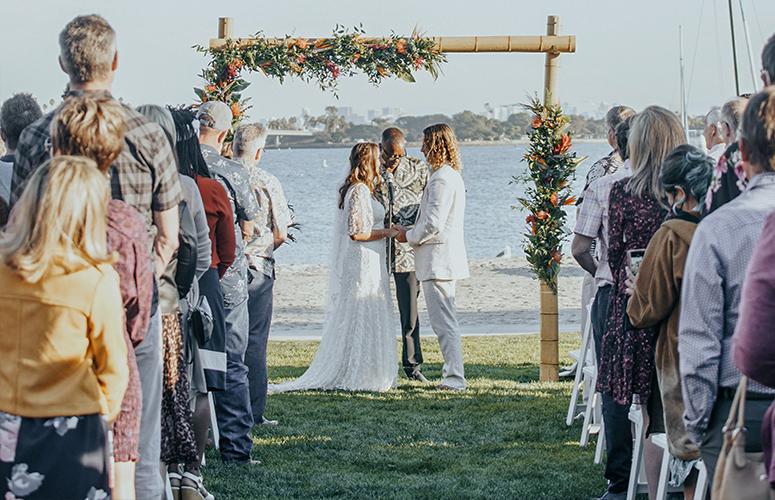The image captures a vibrant beachside wedding ceremony held on a sunny day. At the center of the photo, the bride, dressed in a pristine white dress, stands to the left while the groom, donning a light-colored suit, stands to the right; both have long brown hair. Between them, a man in a floral shirt and glasses, likely the officiant, reads from a book, speaking into a microphone. Above the couple, a decorated archway festooned with red, green, and white flowers frames the scene. The ceremony takes place in front of a picturesque body of water, with a backdrop of sand, distant landmass, and trees, adding to the serene ambiance. Attendees, dressed in colorful attire, including some wearing caps, line both sides of the aisle, intently watching the couple exchange vows on the grassy setting.